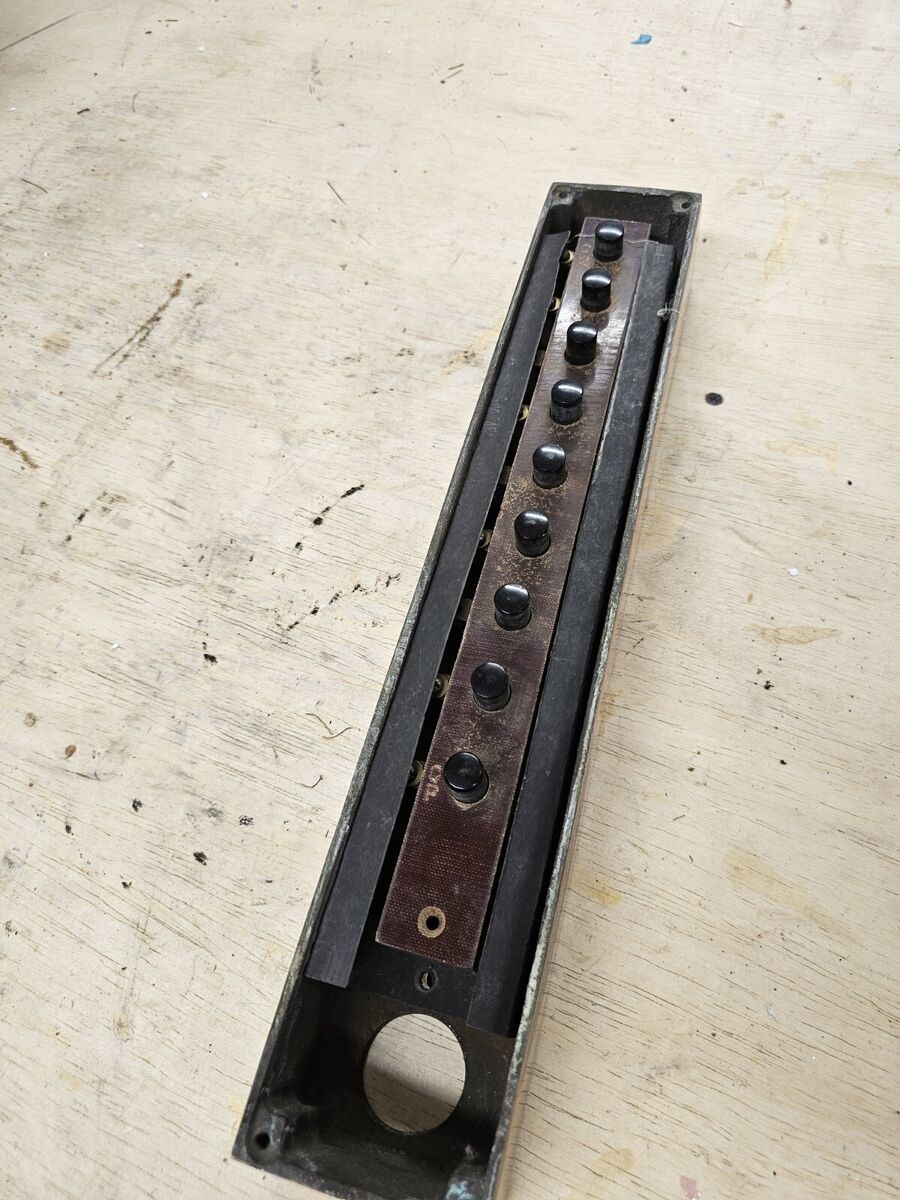A detailed image depicting a white flower with subtle gray tinges and multiple scuff marks in shades of black, gray, and brown. In the foreground, there's a long, black-edged board featuring a hole at one end and a jack input. The board, likely a controller for an electronic device, is also adorned with a series of black buttons.